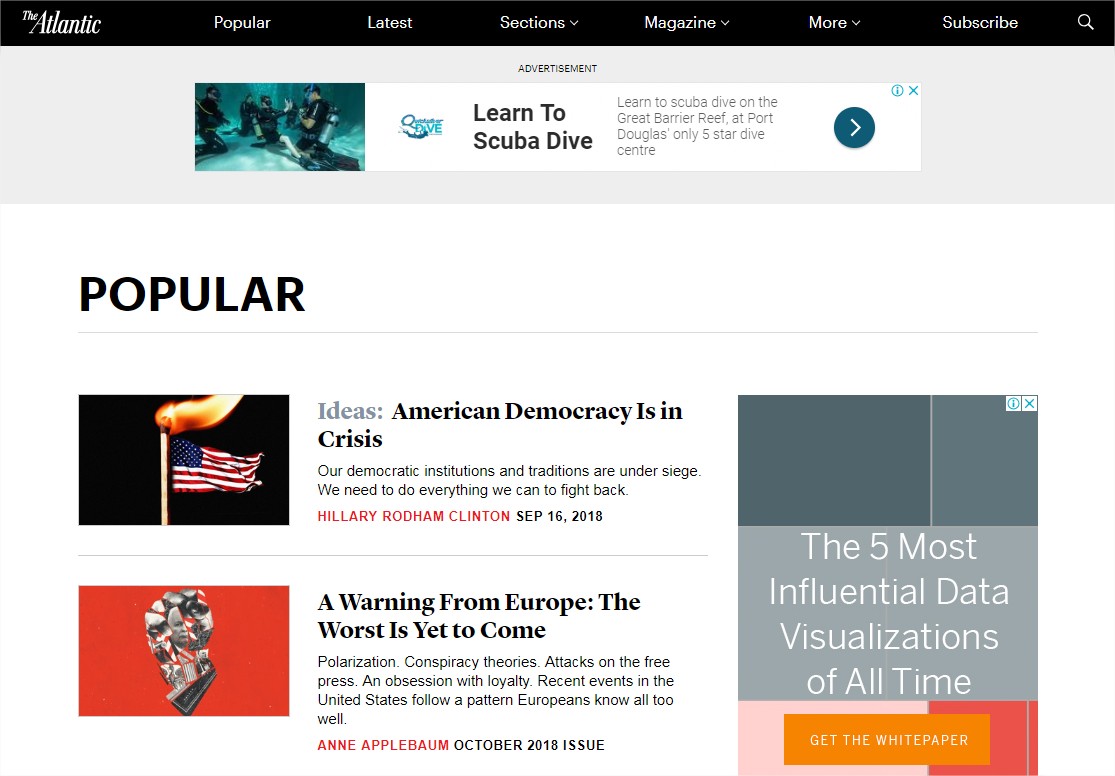The screenshot captures the homepage of The Atlantic magazine's website, renowned for its articles and news. At the top, the navigation bar includes options such as Popular, Latest, various subject sections, and a "Magazine" dropdown with additional choices. The bar also features "More," "Subscribe," and a search icon on the far right. An advertisement banner for scuba diving lessons on the Great Barrier Reef at Port Douglas indicates that the user might be accessing the site from Australia, given the targeted ad's relevance. The page prominently displays popular articles, with a focus on pieces from late 2018. Highlighted articles include "America’s Democracy in Crisis" by Hillary Rodham Clinton, dated September 16, 2018, under the Ideas category, and "A Warning from Europe: The Worst is Yet to Come" by Anne Applebaum from the October 2018 issue. This detailed image captures a snapshot of The Atlantic's popular articles during that specific period.